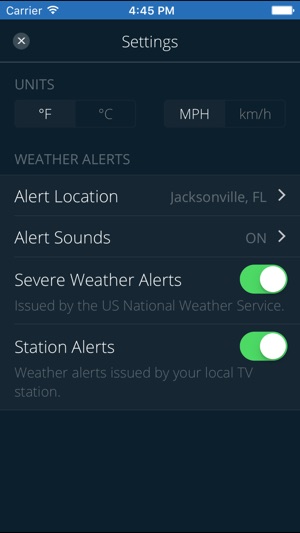A cell phone screenshot captures a settings page for a weather app. The screenshot features a light blue header at the top displaying various icons in white: "Carrier" on the top left, a Wi-Fi signal indicator, the time "4:45 PM" centered, and a battery icon on the top right. The main page has a dark navy blue background with a gray circle containing a white "X" in the top left corner. At the center, the word "Settings" is prominently displayed in white, followed by a horizontal gray line underneath.

The settings shown are specific to weather alerts. The first option, labeled "Weather Alerts" in gray font on the left, lists several configurable items. "Alert Location" is set to "Jacksonville, Florida," with a sideways caret on the right indicating further options. The next item, "Alert Sounds," is marked as "On" in gray, also accompanied by a caret for additional settings. The listing "Severe Weather Alerts," bolded for emphasis, has a subtext reading "Issued by the U.S. National Weather Service" and features an on/off switch set to "On" with a green oval and a white circle indicating its active status. Similarly, "Station Alerts," described as "Weather alerts issued by your local TV station," shows the same active switch configuration.

This detailed breakdown offers a clear and structured view of the weather app's alert settings, emphasizing the functionality and customization options available to the user.